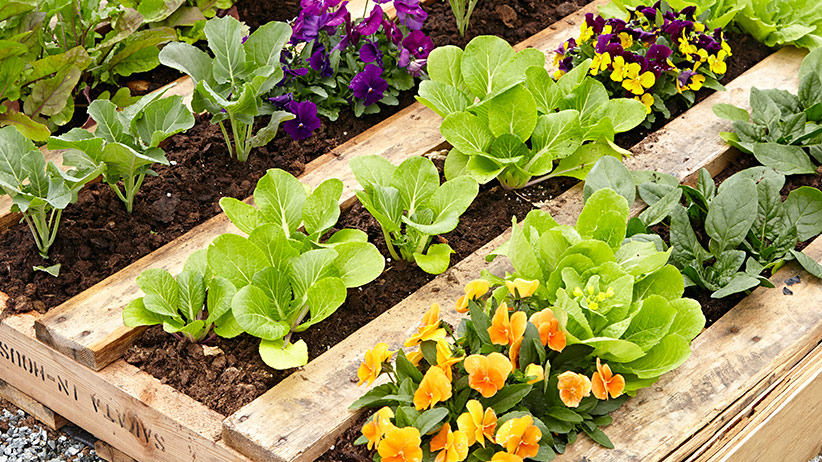The image is a close-up photograph of a raised flowerbed made from a wooden pallet, set outdoors on gravel. The wooden pallet consists of narrow slats filled with brown soil in which various flowers and plants are growing. Dominating the image are colorful clusters of pansies, with vibrant hues of orange, yellow, purple, and deep purple interspersed across the slats. In addition to the pansies, green plants, and possibly some vegetables, contribute to the lush composition. The photo showcases these plants in three distinct rows. In the front of the garden, obscure black letters are visible, though their exact message is unclear. The top and bottom parts of the pallet fade out of focus, underscoring the detailed texture and rich colors of the flowers and foliage that characterize this small, carefully cultivated garden space.